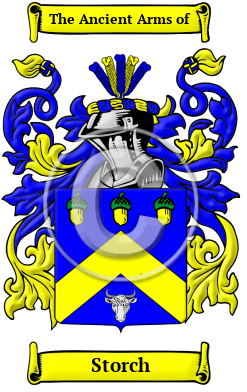The image depicts the coat of arms of Storch. At the top, a gold scroll-like banner reads "The Ancient Arms of." Below, a design in predominantly blue and yellow features intricate curlicues and decorative elements. In the center, a platform showcases a soldier's silver helmet adorned with a floral crown. Surrounding the helmet, three acorns with green caps add detail. Beneath this central section, a white bull's skull is prominently displayed. At the very bottom, a second gold ribbon bears the word "Storch," flanked by yellow orchid-like motifs.